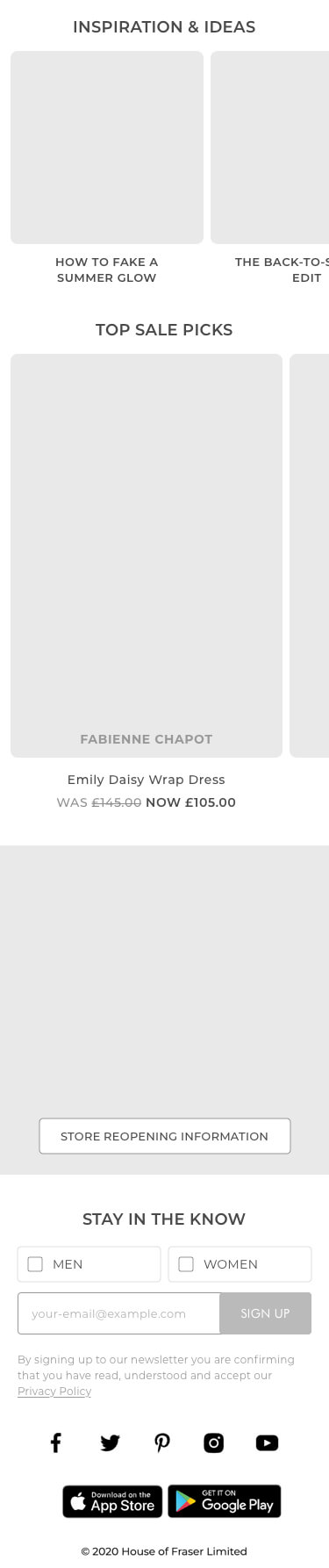This is a screenshot of a webpage displayed with distorted proportions, making all elements appear taller and narrower than usual. The background is white. At the top center, there is a grey, all-caps heading, "INSPIRATION & IDEAS," featuring an ampersand. 

Below this header, there are two adjacent rectangular tiles with light grey backgrounds and slightly rounded corners. The left tile is fully visible, while the right tile is only partially visible, cut off by the edge of the frame. Both tiles are labeled with smaller grey all-caps text. The first tile on the left is labeled, "HOW TO FAKE A SUMMER GLOW," and the second tile, which is partially obscured, reads "THE BACK TO DASH EDIT," with part of the text cut off.

Further down, there is a centered line of all-caps dark grey text that reads, "TOP SAIL PICS." Beneath this text, there is a larger light grey rectangle with slightly rounded corners. Centered at the bottom of this rectangle is medium grey all-caps text that says, "FABIEN CHAPEAU." To the right of this rectangle, separated by a narrow strip of white space, there is another similar rectangle that is mostly cut off by the edge of the frame.

Below the first large rectangle, there is non-all-caps medium grey text that reads, "Emily Daisy Wrap Dress." Underneath this line, there is light grey text slightly to the left that was originally priced at £345, crossed out. To the right of this crossed-out price, in black text, is the new price, "Now £105."

Finally, there is another rectangle beneath this section, accompanied by additional text that also follows the same design style.